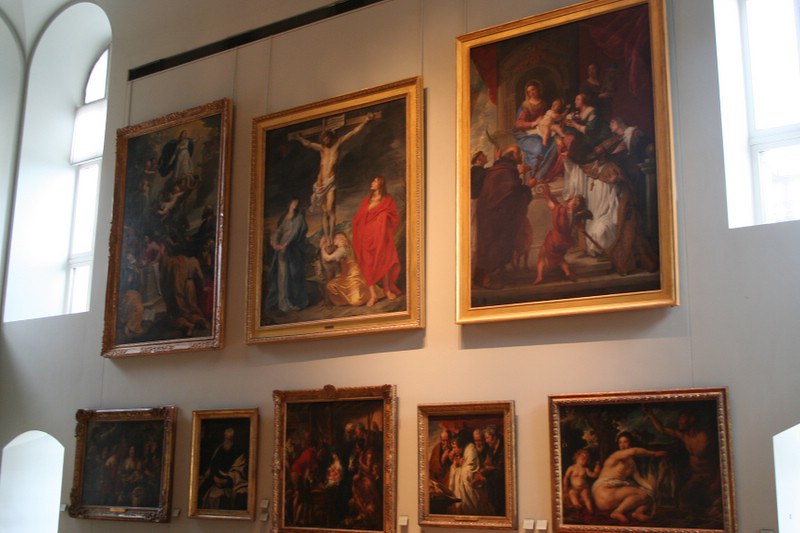The photograph captures a section of a white wall inside a spacious hall, possibly part of a museum or a private art collection. The hall features arched windows that frame the collection and allow natural light to illuminate the display. Eight framed oil paintings, arranged in two rows, dominate the wall. The top row consists of three larger paintings, while the bottom row displays five smaller ones. All frames are crafted from gold-painted wood, adding a touch of elegance to the historic artwork. 

The paintings depict various scenes from the life of Jesus Christ, rendered in a romantic classical style. The centerpiece of the collection shows Jesus crucified on a cross, with women at his feet in an emotional tableau. Flanking this central piece, one painting portrays the Adoration of the Magi, with the three kings visiting baby Jesus, while another also highlights the nativity scene. Other paintings feature cherubic infants, women draped in white cloths, and figures in vibrant, historical robes. Each painting, rich in detail and historical biblical context, reflects the elegance and reverence typical of the era they represent.